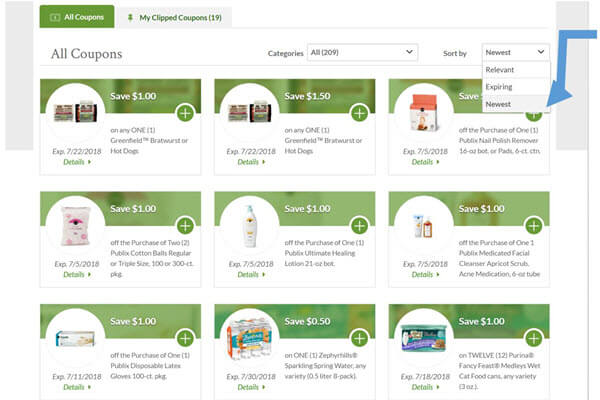The image depicts a screenshot of a web search result, specifically from a coupon website. The background is predominantly white, providing a neutral canvas that makes the varying shades of green for the tabs stand out. In the top left corner, a moss-green tab is labeled "All Coupons" in white text. Adjacent to it, a gray-colored tab reads "My Clipped Coupons," indicating that 19 coupons have been clipped.

Beneath these tabs, the main section is organized into three distinct rows filled with various coupons. The coupons offer discounts ranging from $0.50 to $1.50 off on different products. Notably, the displayed coupons include items such as toilet paper and Zephyrhills bottled water. The interface suggests this might be a Publix supermarket website.

A prominent blue arrow on the right-hand side of the screen points downward towards a toolbar. This toolbar features clickable options, and the user has selected the option labeled "Newest."